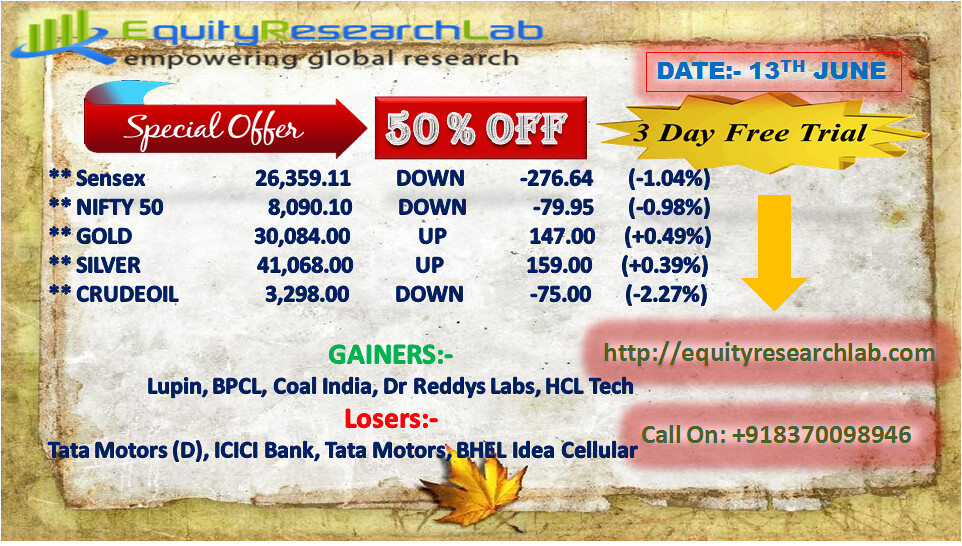The image is a colorful advertisement presented as a screenshot of a computer screen. The background features a variegated pea-green design. In the upper left corner, green and blue text prominently displays "Equity Research Lab," with the tagline "Empowering Global Research" in black text below. Adjacent to this, a blue 'Q' encircles four ascending green bar graphs. 

A striking red banner beneath the tagline announces a "Special Offer" with an arrow pointing to a bold red rectangle proclaiming "50% off." The advertisement also includes a date in the upper-right corner, "June 13th," and offers a three-day free trial.

Dominating the center are key financial metrics: 
- Sensex: $26,359.11
- Nifty 50: $8,090
- Gold: $30,084
- Silver: $41,068
- Crude Oil: $3,298, down by $2.76

The lower left-hand side features "Gainers" in green text and "Losers" in red text. On the right-hand side, it lists the website "equityresearchlab.com" and a contact number, area code 918-370-0989. The entire advertisement is visually organized to highlight stock market information and promotional offers, suggesting its purpose as a stock research and financial advisory tool.